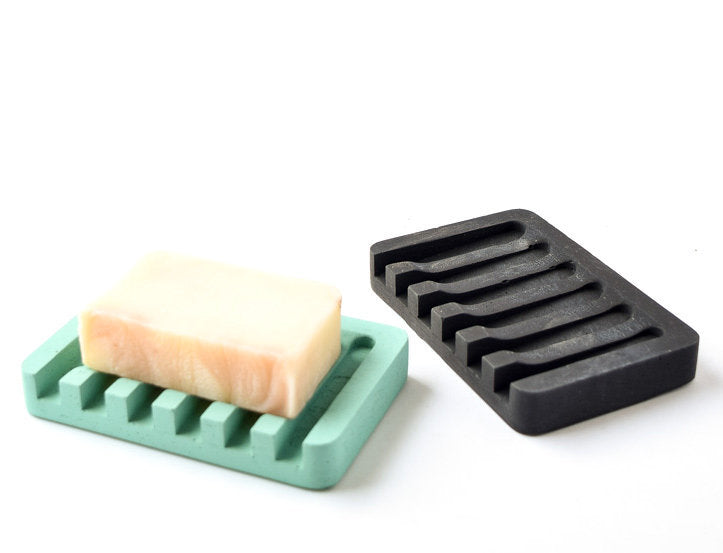The image displays two soap dishes set against a stark white backdrop, creating a clean, professional product presentation. Both dishes share the same rounded rectangular design, each slightly larger than the soap bar they hold. The soap dishes feature six grooves or slits intended for drainage. The left soap dish is a light mint green, featuring a white ivory soap bar centrally placed, fitting neatly within the grooves. The soap bar appears rectangular with a slightly squared-off shape and a marbled texture of white and tan. The dish on the right is black and shows signs of use with some white or gray residue likely from previous soap. Both dishes are thin, with an approximate thickness of an inch, and their curved edges contribute to a streamlined appearance. The well-lit image has a minor drop shadow effect, enhancing the product's minimalist aesthetic against the pristine white background.